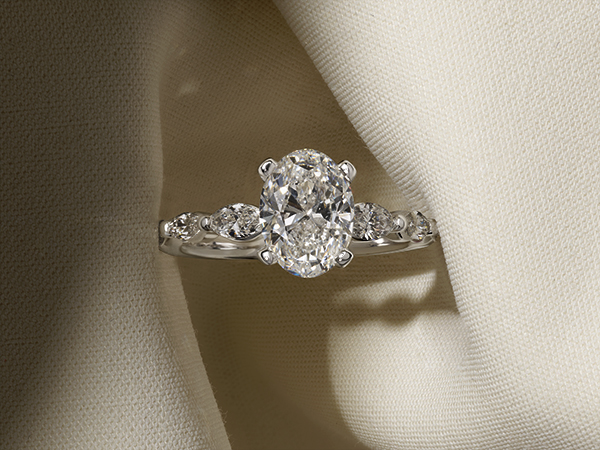This close-up photograph captures a stunning, silver diamond engagement ring elegantly nestled within the folds of a cream-colored linen or cloth, giving off a textured, burlap appearance. The ring features a prominent, oval-shaped central diamond held securely by four prongs, surrounded by additional smaller diamonds along the band. The setting, likely white gold or platinum, accentuates the sparkle and clarity of the diamonds. The cloth, appearing brighter on the right and more shadowed on the left, showcases the ring in a perfectly centered position, creating a harmonious balance in the composition. Shadows cast by the ring add depth, emphasizing the pristine, lustrous quality of the jewelry. The overall scene is beautifully understated, highlighting the ring's brilliance and fine details, making it an ideal representation of a timeless piece of jewelry.